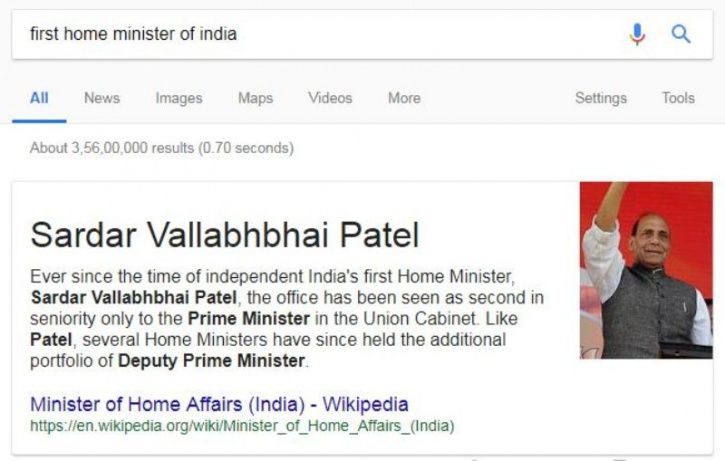The image is a detailed screenshot of a Google search result page. At the very top, the search query typed into the search bar reads, "first Home Minister of India." The familiar Google interface presents various navigational tabs under the search bar, including "All," "News," "Images," "Maps," "Videos," and "More." To the right side, options for "Settings" and "Tools" are visible. 

On the left side, just below the tabs, the page indicates the total number of search results found, approximately 3 billion, and the time taken to retrieve them, 0.7 seconds (in parentheses). The primary answer to the search query is prominently displayed: "Sardar Vallabhbhai Patel," accompanied by a photograph of him on the right side of the page. The result provides an immediate and concise response to the query, illustrating Google's efficiency in delivering high-volume information quickly.